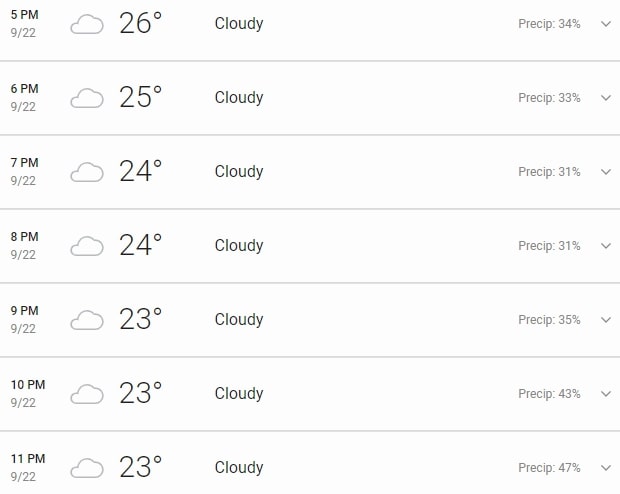A detailed weather forecast is displayed in this image. The forecast spans from 5 p.m. to 11 p.m. on the 22nd of September. The date format suggests it aligns with the UK convention, where the day precedes the month. 

For each hour within this period, the forecast indicates consistent cloudy conditions. Temperatures show a gradual decline from a high of 26°C at 5 p.m. to 23°C by 11 p.m. Specific hourly temperatures are as follows: 
- 5 p.m. - 26°C
- 6 p.m. - 26°C
- 7 p.m. - 24°C
- 8 p.m. - 24°C
- 9 p.m. - 23°C 
- 10 p.m. - 23°C 
- 11 p.m. - 23°C

In addition to temperature and cloud coverage, the forecast provides precipitation probabilities, ranging from 31% to 47%. The precise values of precipitation percentages for each hour are not detailed. Though the source of the weather forecast is not specified, it gives a comprehensive hourly overview for planning outdoor activities or commutes.